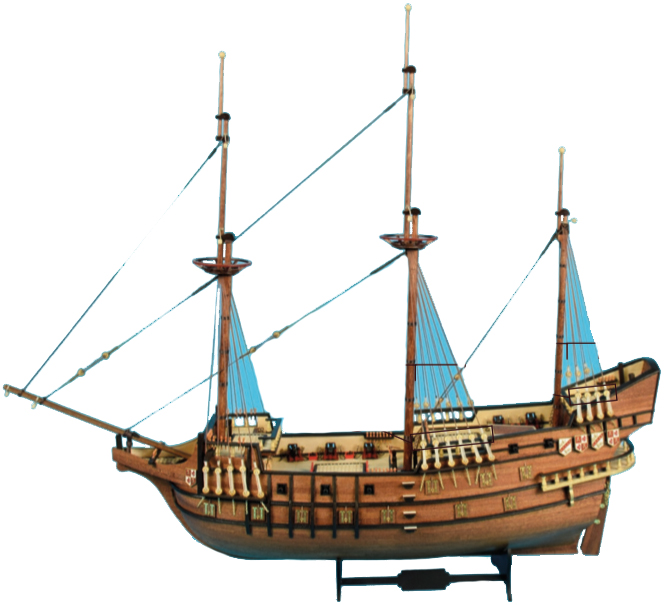This photo showcases a detailed model of an older ship, reminiscent of vessels from the 1600s to colonial times. The side profile reveals a large wooden vessel with multiple floors, emphasized by layers of cannon ports and windows on the deck. It features three prominent masts, the two at the front topped with crow's nests. Elegant blue sails are draped from the masts, secured with thick ropes extending to the front and back of the ship. The ship, propped on a little black stand against a white or transparent background, has an intricate design highlighted by light wood finishes with darker accents on the lower hull. Ornate railings, possibly made of balsa wood, line the sides, and small cannons or cannonballs are positioned along the deck's edges. The masts are adorned with small flags and turquoise blue elements, and midway up the masts, a bowl-like feature helps hold the structure together. The meticulous craftsmanship and vibrant details suggest it could be a high-quality toy or a collectible model ship.